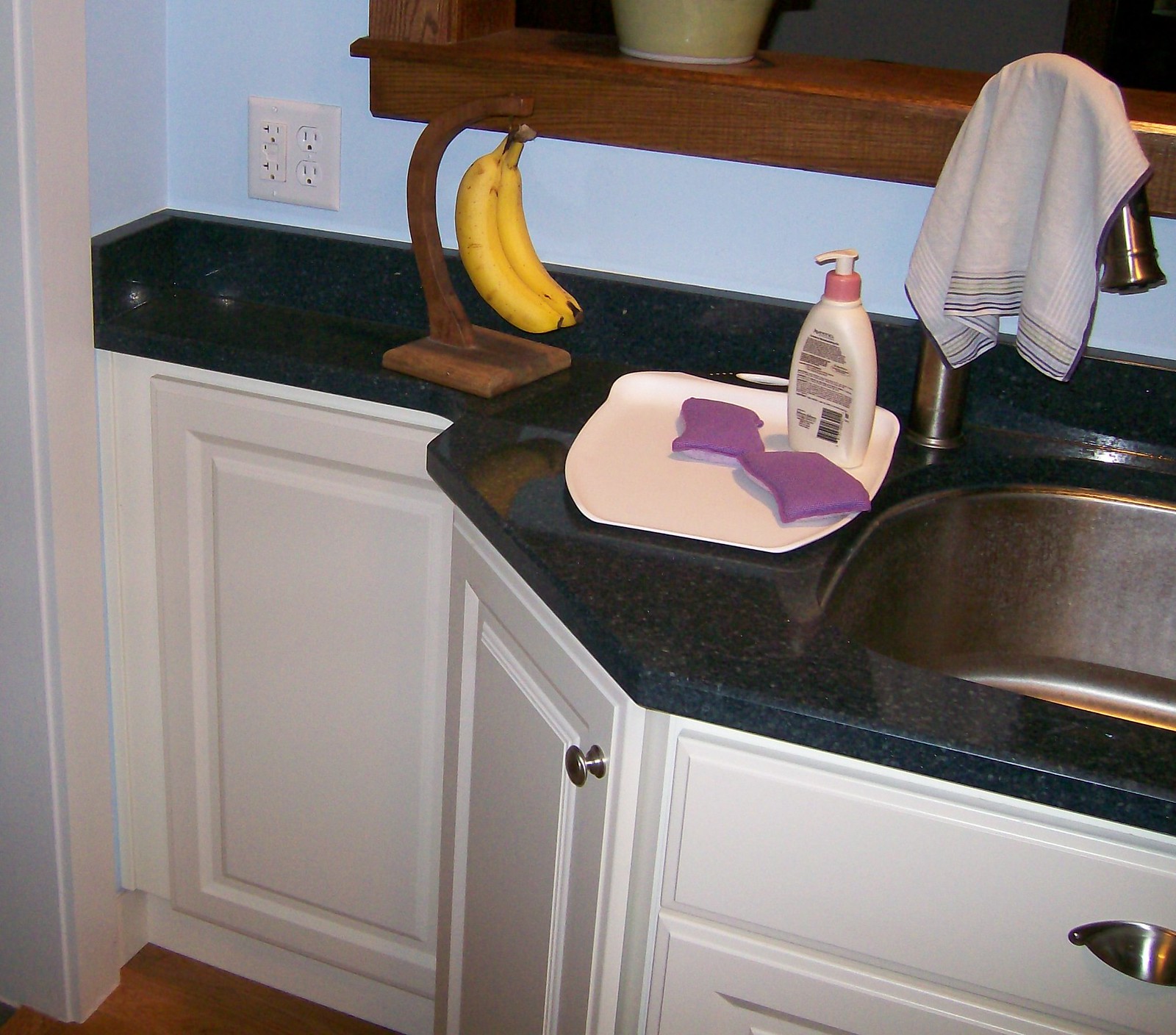The image captures a brightly lit kitchen, focusing on both the countertops and portions of the cabinetry. The bottom half of the image displays four distinct drawers. On the bottom left, there is a long rectangular drawer with a wooden, white-colored front, though its handle is not visible. To the right of this, in the bottom middle section, a diagonal-angled drawer is visible, featuring a silver metal handle at its top right corner. Further right, in the bottom right corner of the image, are two horizontally-aligned drawers stacked vertically. The visible handle on the central drawer is silver and reflective.

In the top half of the image, the countertop is prominently displayed. On the top left, the kitchen's light blue wall features a white outlet panel with four outlets; the two on the left are square-shaped while the two on the right are hexagonal. Situated in the middle of the countertop is a bunch of bananas hanging from a brown banana holder. To the right, part of the sink is visible, adorned with a gray rag draped over it. Immediately to the left of the sink sits a white bottle of lotion, completing the array of items on the countertop.